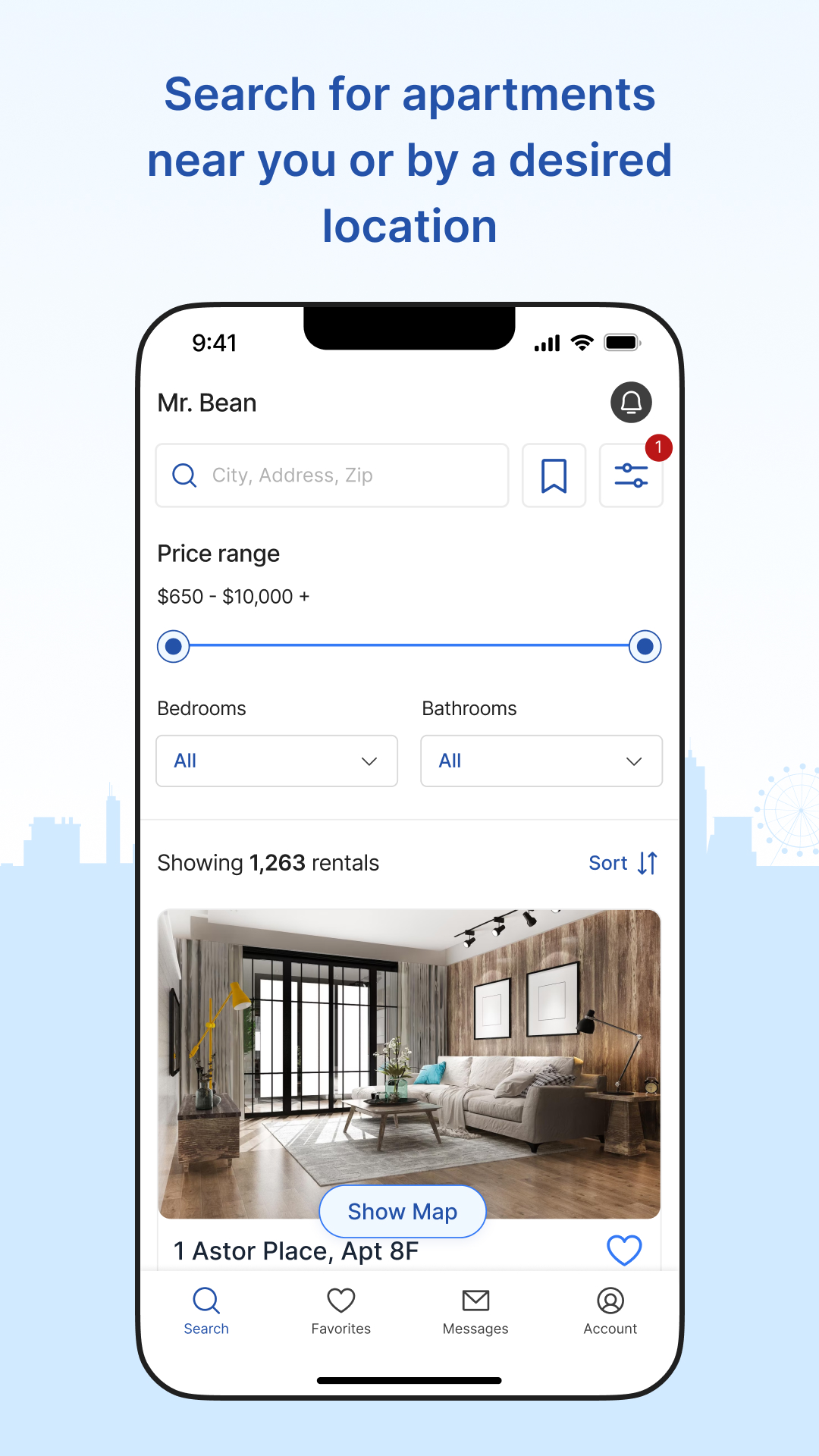This is a detailed screenshot of a mobile phone app designed for searching apartments. The app's main interface prominently displays a search bar labeled "Search for apartments near you or by desired location," with a set of customizable filter options and a bookmark tab positioned nearby. The filters allow users to specify their search criteria based on price range, from $650 up to $10,000, and to select the number of bedrooms and bathrooms needed.

The results page indicates a total of 1,263 available rentals matching the applied filters. The first listing in the search results features an inviting photograph of a well-appointed living room. The room boasts a stunning faux wooden accent wall and a polished wooden floor. A pristine white couch, complemented by two decorative pictures hanging above, anchors the space. The room is bathed in natural light streaming through large, bright windows supplemented by elegant French-style doors that likely lead into an adjoining room.

The living room is furnished with a set of two tables—a central coffee table and another table on the left side, possibly intended for a television. The overall ambiance is enhanced by stylish lighting fixtures, creating a warm and welcoming atmosphere.

Additionally, the app interface includes a useful map icon for visualizing apartment locations, along with a series of functional tabs such as Search, Favorites, Messages, and Accounts, providing a comprehensive and user-friendly experience for prospective renters.